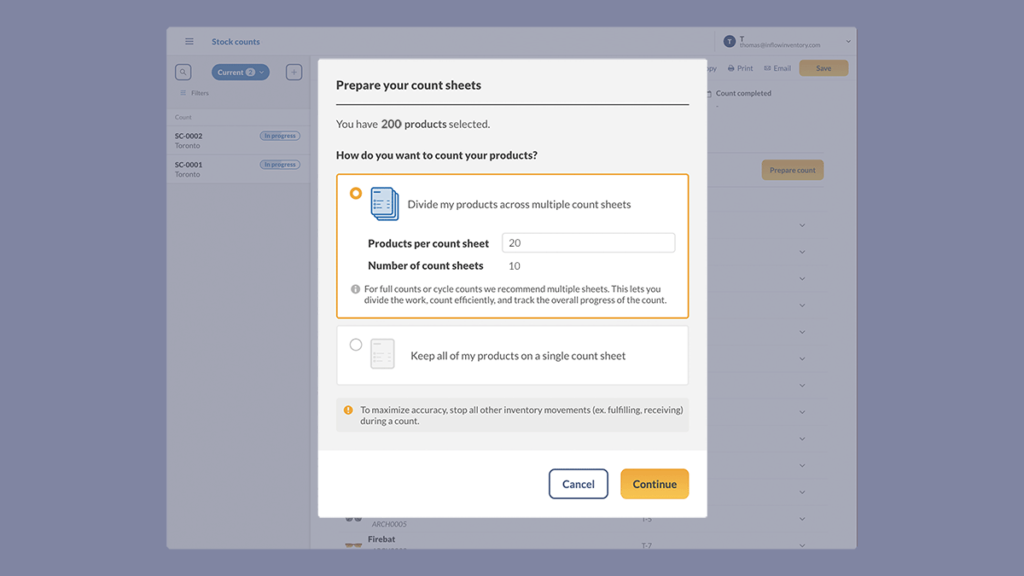A screenshot from a stock management site shows a detailed interface for managing inventory counts. At the top, the title "Stock Counts" is displayed prominently. Below it, a blue rectangular bar with rounded edges features the word "Current" in white text and the number "2." 

In the background, two different stock counts, "SC0002" and "SC0001," are visible but grayed out due to a central pop-up window. The pop-up's title, in black text, reads "Prepare Your Count Sheets." Beneath this, a message indicates, "You have 200 products selected." Another line in black text poses the question, "How do you want to count your products?" 

The user has chosen the option to "Divide my products across multiple count sheets," specifying 20 products per sheet and a total of 10 count sheets. At the bottom of the pop-up are two buttons: a yellow "Continue" button with black text and a "Cancel" button.